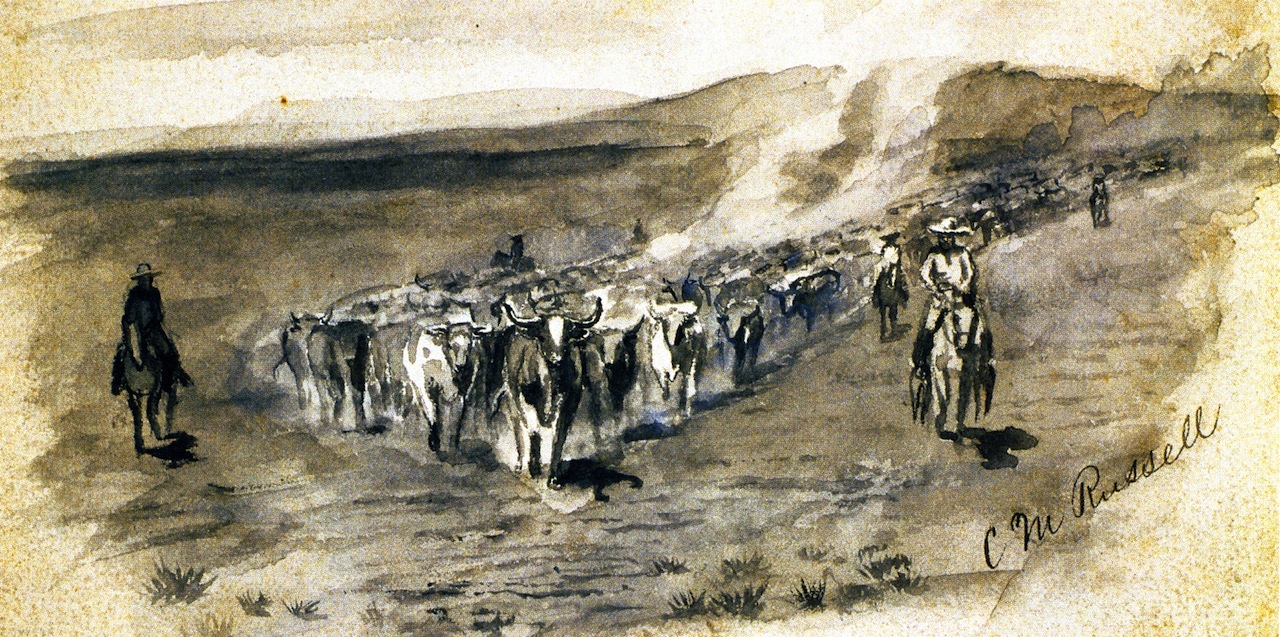This is a detailed painting by C.M. Russell, whose signature can be seen in the lower right corner. The artwork portrays a dynamic scene of a cattle drive across a vast desert landscape. In the foreground, a large herd of cattle is being herded by men on horseback, who are diligently guiding the animals. The painting, with a watercolor-like quality, uses mostly black ink on a parchment-colored paper. Sparse bushes dot the arid terrain, and a substantial ring of dust clouds rises behind the moving herd, adding to the sense of motion. Faded mountains loom in the distance under a clear, bright sky, completing the expansive and rugged scenery.